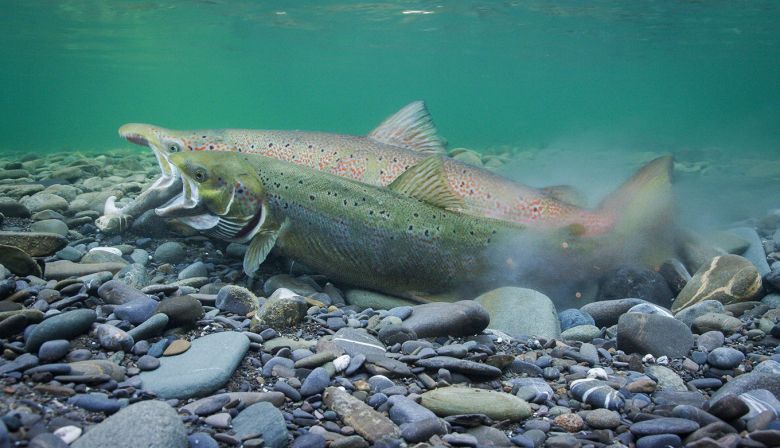This underwater photograph vividly captures the serene life below the water surface, highlighting two fish resting among a bed of smooth gray rocks of various shapes, sizes, and hues, interspersed with occasional seashells. The clear, greenish-blue water above reflects light, adding a shimmering effect that accentuates the tranquil setting. In the foreground is a greenish-yellow fish with small dots, its mouth wide open, yet not as expansive as the larger fish behind it, which displays a pinkish tone with tiny dots. Both fish, resembling trout or salmon, seem poised in an open-mouthed stance, possibly hunting for food or engaging in a behavior that stirs up a dusty mess, suggesting a dynamic underwater interaction against a backdrop of colorful, reflective water.